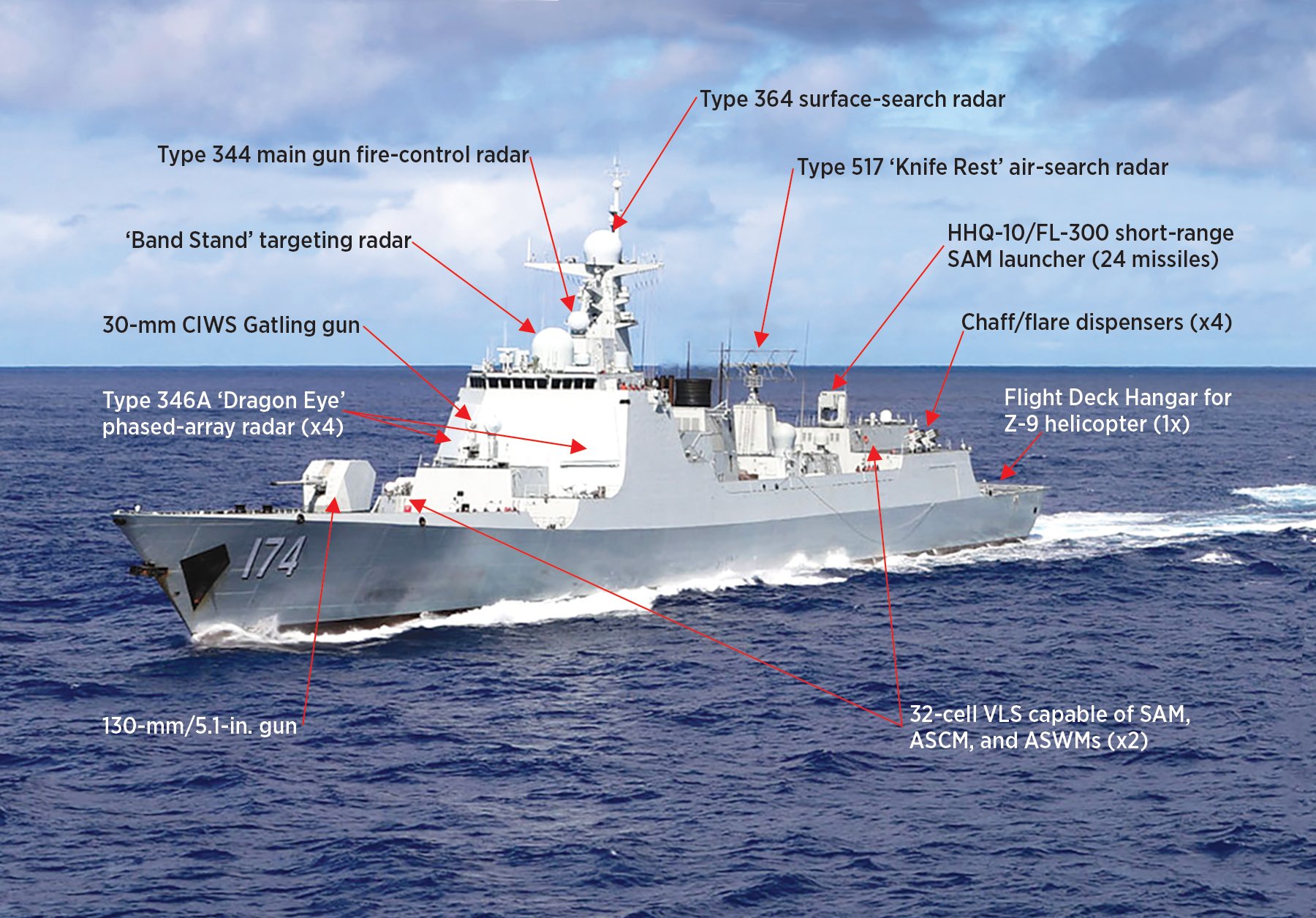This is a detailed poster image of a naval battleship, prominently numbered 174 on its front side, navigating the ocean waves. The ship features a combination of white and gunmetal hues, and only the left side of the vessel is visible. Multiple red arrows point out and label various parts of the ship. At the front, there's a 130mm / 5.1-inch main gun, with a 30mm CIWS Gatling Gun above it, and several radar systems atop the structure, including the Type 346A Dragon Eye Phased Array Radar and the Bandstand Targeting Radar. Midship, a 32-cell VLS is capable of launching various surface-to-air and anti-ship missiles. Further back, highlighted elements include the Type 344 Main Gunfire Control Radar, the Type 364 Surface Search Radar, the Type 517 Knife Rest Air Search Radar, and an HHQ-10-FL300 Short Range SAM Launcher with 24 missiles. The ship also houses the shaft flare dispensers (x4) toward the rear, and a flight deck hanger designed for a Z-9 helicopter.